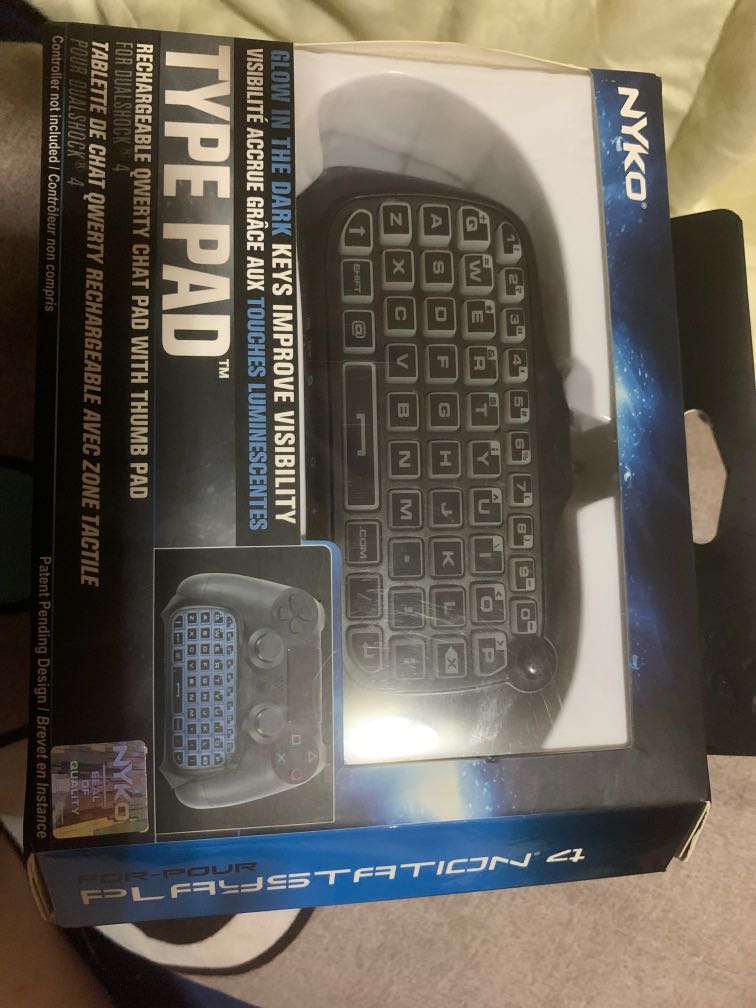In the image, we see a Nyko Type Pad prominently displayed in its packaging. The package, oriented vertically, showcases the sleek keyboard-like Type Pad with clearly visible keys arranged in a QWERTY layout for easy typing. The keys are designed to glow in the dark, enhancing visibility in low-light conditions, as indicated in both English and another language on the packaging.

The packaging itself is predominantly black with a clear plastic window, allowing you to see the product inside. The front of the package features bold white lettering that reads "Type Pad" and highlights the product's rechargeable function. Additionally, it describes the Type Pad as a "Rechargeable Chat Pad with Thumb Pad," emphasizing its user-friendly design for efficient communication.

Accompanying the main image of the Type Pad is a smaller pop-up image on the right side, showing the Type Pad in use. This illustration provides a better understanding of its practical application. Behind the package, there is a beige background with a circular white element featuring a black center, adding a contrasting visual detail.

At the top of the package, there is a small tag with a hole, designed for easy hanging in retail stores. This thoughtful detail ensures the product can be conveniently displayed and accessed by customers. Overall, the image and packaging provide a comprehensive view of the Nyko Type Pad, highlighting its key features and usability.